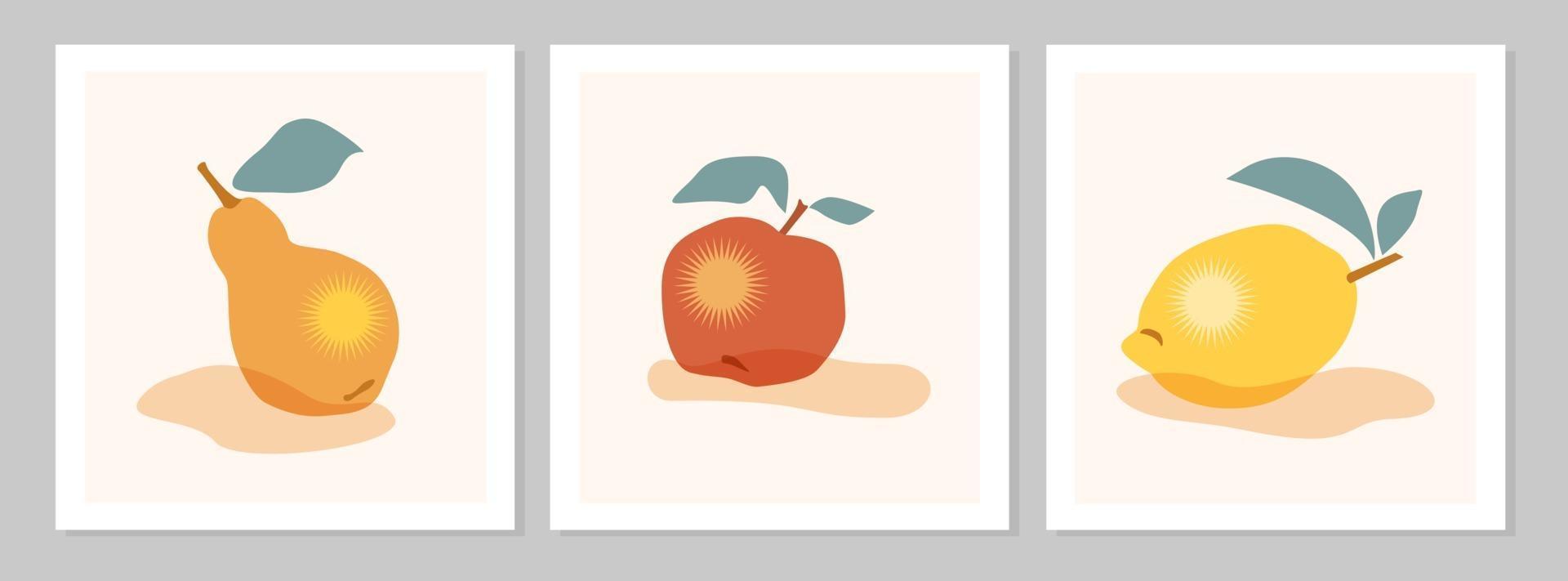The image features a series of three square computer-generated illustrations of fruits, arranged horizontally and presented in landscape mode. Each illustration is framed by a white border, and the background within each frame is a very pale peach color. The fruits are laid out on a gray background, possibly representing a cardboard-like sheet.  

From left to right, the first illustration depicts a pear with a light orange-yellow tint, accompanied by a brown stem and a green leaf. The pear's stem faces the upper left-hand corner. The second illustration, in the center, shows a bright red apple with a yellowish reflection symbolizing light. This apple has a dark red stem and two green leaves, with the stem pointing to the upper right-hand corner. The third illustration on the right features a yellow lemon, also with a light reflection symbol, a brown stem, and two green leaves. The stem of the lemon is oriented mostly to the right while slightly upwards. All three fruits have a stylized shadow effect rendered in black. The detailed and colorful representations of the pear, apple, and lemon are the focal points of the image.